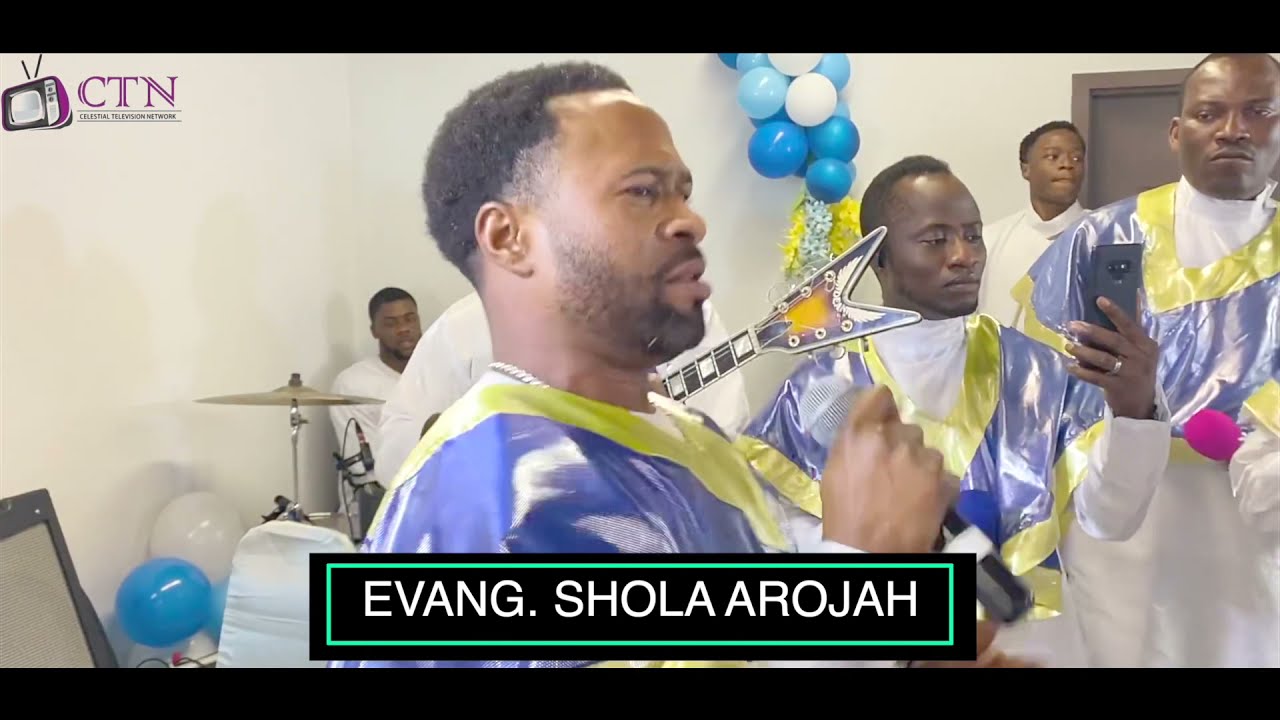The image captures a group of black individuals seemingly in a church setting, with three of them donned in white robes accessorized with blue and yellow V-shaped stoles. The central figure, holding a microphone and a cell phone, appears to be the main focus. He is flanked by other men, including one with black hair and a beard, and another peering over at the cell phone. In the background, one person sits at a drum set partially obscured by the foreground figures. To the right, another man looks away from the central action. The backdrop features a white wall adorned with blue, light blue, and white balloons, a wooden door on the right, and a left-side logo of a TV with "CTN" in pink font. Beneath this, partially legible text trails off. Positioned at the bottom, within a black rectangle framed by a gray-green border, it reads "EVANG. Shola Araja" in white letters.